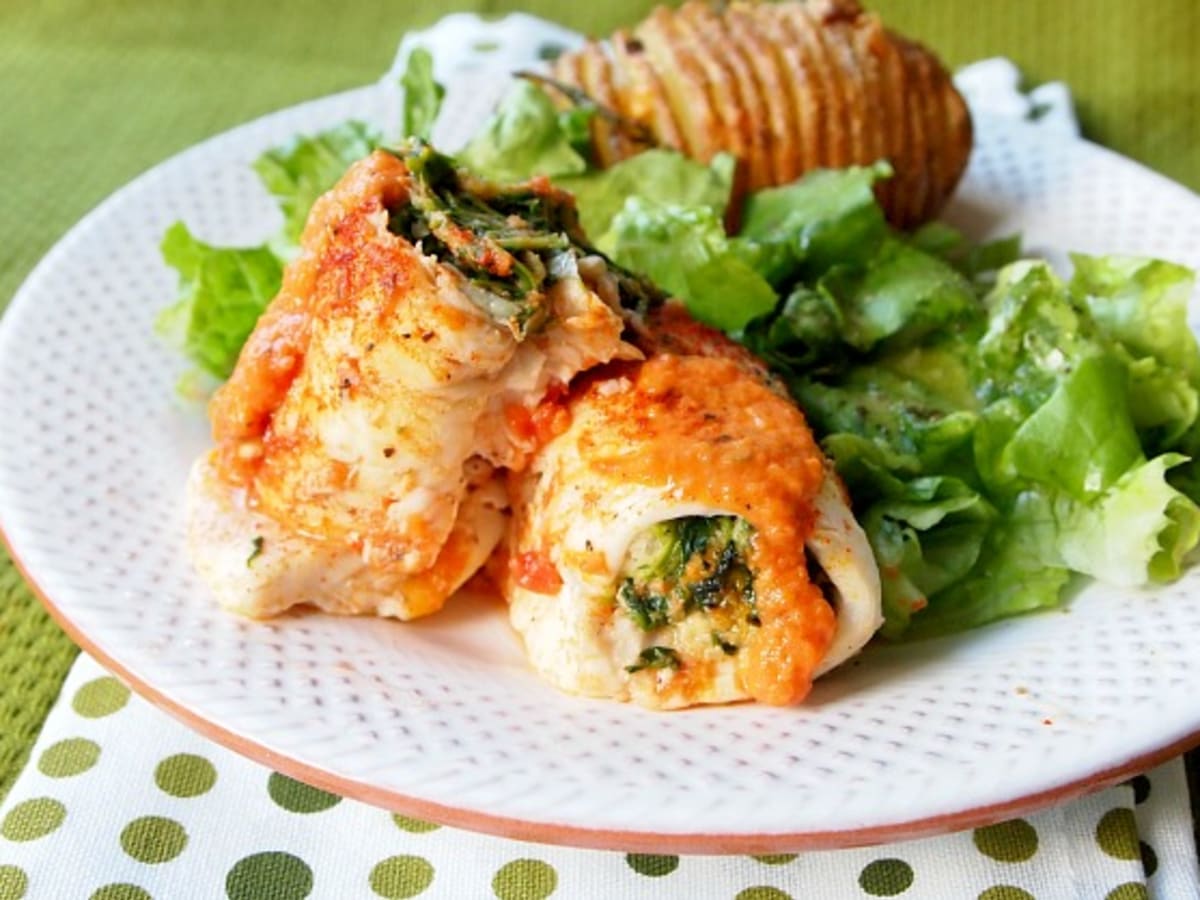In this image, a large white ceramic plate with a textured, dimpled edge and a brownish-red border takes up most of the frame. The plate is set on a white placemat featuring varying shades of green dots, which in turn rests on a woven green tablecloth. The right portion of the plate is slightly cut off from the view.

The plate holds an appetizing arrangement of food. There is a bed of green lettuce, possibly dressed, spread across the plate. In front of the lettuce, closer to the camera, are two stuffed food items resembling chicken or a white meat dish, each piece positioned differently – one leaning forward and the other sideways. The stuffing inside these rolls appears to be a mixture of green vegetables, such as broccoli, and possibly melted cheese. An orangey sauce or melted cheese adds a crispy, slightly browned texture on top. Additionally, toward the far end of the plate, there is a fanned baked potato with fine slices cut throughout its entire surface.

The combination of textures and minor details, like the dotted pattern on the plate's edge and the carefully arranged layers of the potato, adds a sense of homemade culinary artistry to the scene.